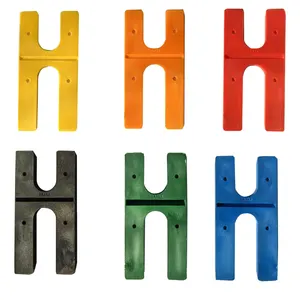Here is an image showcasing six colorful, H-shaped plastic pieces arranged on a white background. These pieces are aligned in two rows, each containing three objects. In the top row, the first H-shaped object is yellow, followed by an orange one in the middle, and a red one on the right. In the bottom row, the sequence begins with a black H on the left, continues with a green one in the middle, and ends with a blue H on the right. Each of these pieces features four small circular indentations, with two near the top arms and two near the bottom arms of the H shape. Additionally, there is a noticeable crease or hinge about three-quarters of the way up the objects, suggesting they might fold, although the top portion would be shorter than the bottom. Subtle highlights on the surfaces give the objects a shaded appearance, enhancing their vibrant colors. There is no text in the image, leaving the purpose of these H-shaped pieces open to speculation.